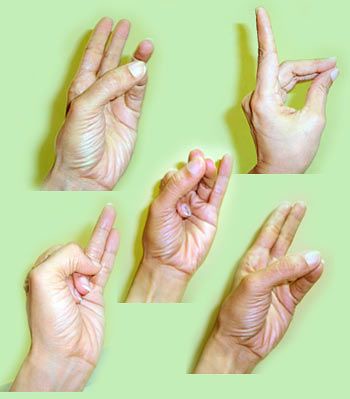The image depicts a series of five left hands arranged against a green background, each performing different hand gestures that are likely related to sign language. The hands are displayed in a symmetrical fashion with four in the corners and one in the center. 

- **Top Left:** The thumb touches the pinky finger, creating a circular form with the other fingers extended.
- **Top Right:** The hand forms a gesture where the thumb touches all fingers except the index finger, which is extended upwards.
- **Center:** The main (or index) finger is pulled down, with the thumb touching the middle and ring fingers.
- **Bottom Left:** The first two fingers are folded under the thumb, while the last two fingers (ring and pinky) are extended upwards.
- **Bottom Right:** The thumb touches the last two fingers (ring and pinky) again, similar to a different position shown previously.

The hands are tan in color, emphasizing clear contrast against the green background, and each gesture appears to be part of a structured representation, possibly indicating different letters or words in sign language.